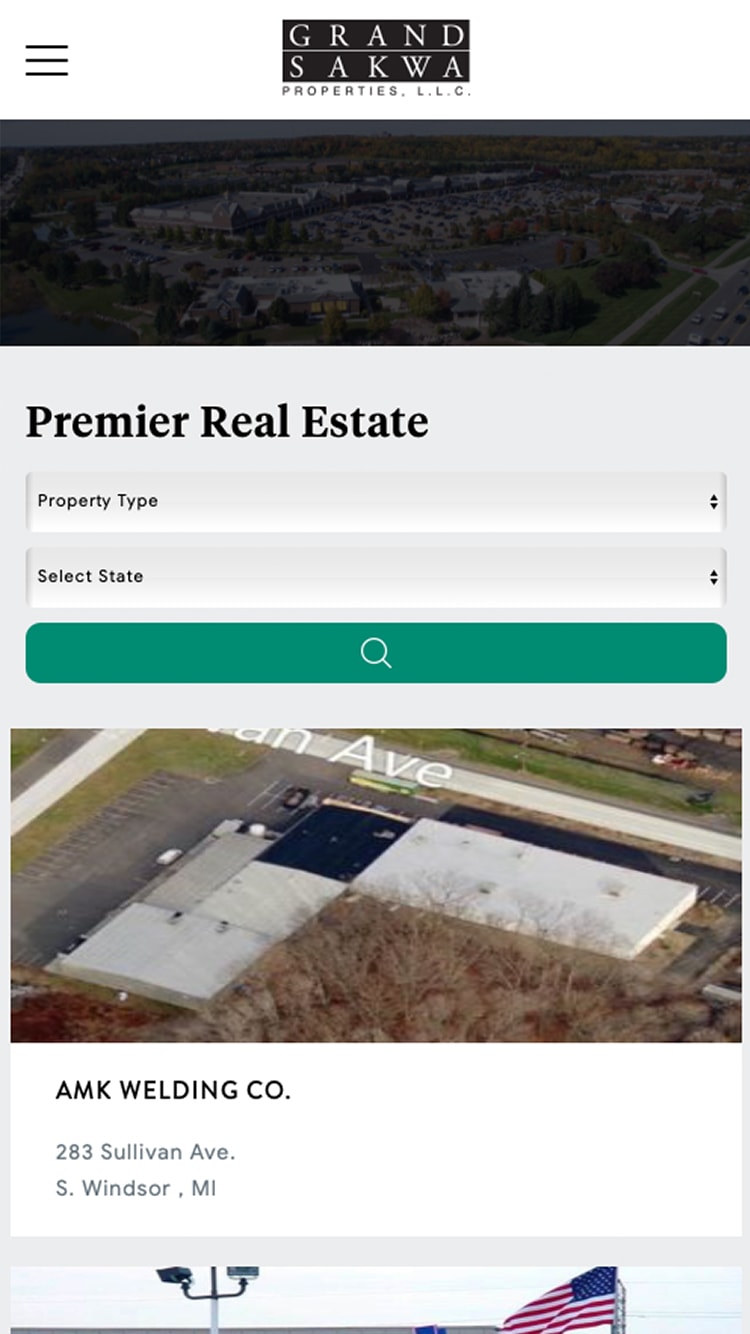The image captured from a real estate website appears to be displayed on a mobile device, featuring a vertically-oriented, rectangular shape. The top inch of the screen features a black border. 

On the left side, there is a white border that contains three stacked black lines. Centered below this, there is a black rectangle with the word "Grand" written in white text, followed by a line and then "Sakwa" (spelled S-a-k-w-a). Below this, in black letters, it says "Properties L.L.C."

Underneath this section, there is a hazy image depicting a development property with buildings spread across the center portion of the image from left to right. The surrounding area is filled with greenery and there’s a sliver of sky at the top.

Beneath the image, a light blue border appears on the left-hand side with bold black letters stating "Premier Real Estate." Directly below this, there is a search tab labeled "Property Type" and another one below it that reads "Select State." Further down, there is a long, rectangular teal button featuring a white search icon in the center.

Additionally, there is another image showing the top of a building, extending from about an inch from the left corner, nearly an inch from the top, and to about an inch from the right edge. Surrounding this building are patches of grass and trees.

Below this, in a white bordered section, there is black text reading "AMK WELDING CO." in capitalized letters. Below that, in smaller black text, it states "283 Sullivan Avenue, S. Windsor, MI." Across the bottom of the image, a blue border is visible with a portion showing a lamp post two inches from the left corner and an American flag on the right side.